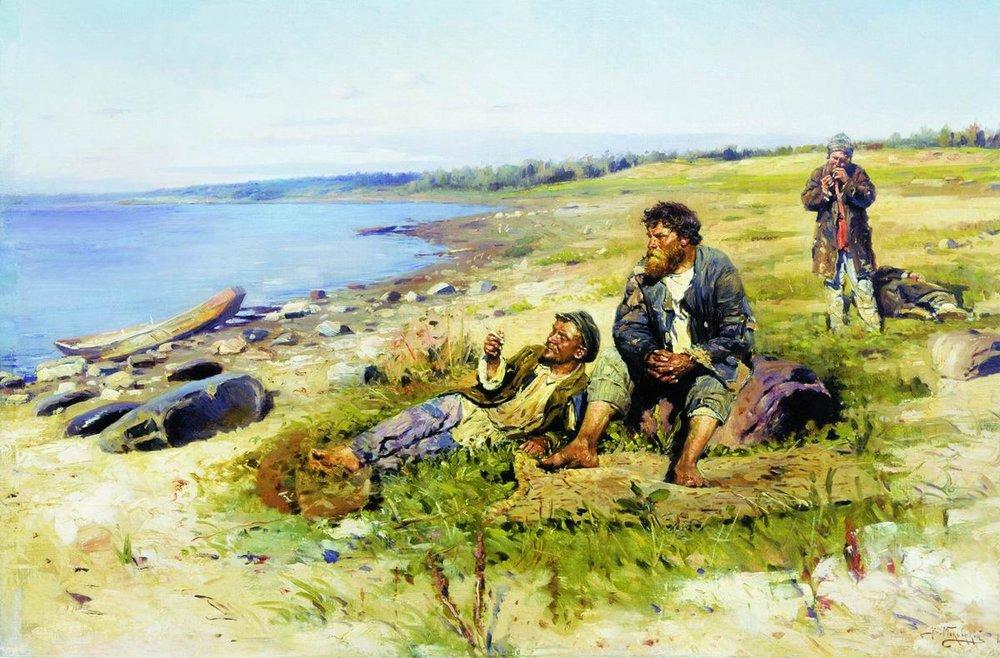This detailed painting depicts a serene outdoor scene by the shore of a large lake. The setting showcases three men resting on a patch of straggly grass just above the rocky shore. The man in the foreground is reclining against a rock or log, propped up by his elbow, casually smoking a cigarette. He is barefoot, dressed in shabby clothing, including a brown scally cap, a torn brown jacket, a white shirt, and soiled blue-gray pants. Next to him, seated on a rock, is a heavier man with a beard, wearing a wrinkled or torn gray jacket over a white shirt and gray pants that are rolled up past his calves, revealing dirty feet. Behind them, a third man stands, his gaze cast downward as he lights a cigarette. He is clad in a long, tattered brown coat over ragged gray pants. A boat rests on the rocky shore, adding to the tranquility of the scene. The background features a vibrant blue sky scattered with clouds and a calm expanse of blue water to the left, contrasting sharply with the green grass and earthy tones of the men's attire and surroundings.